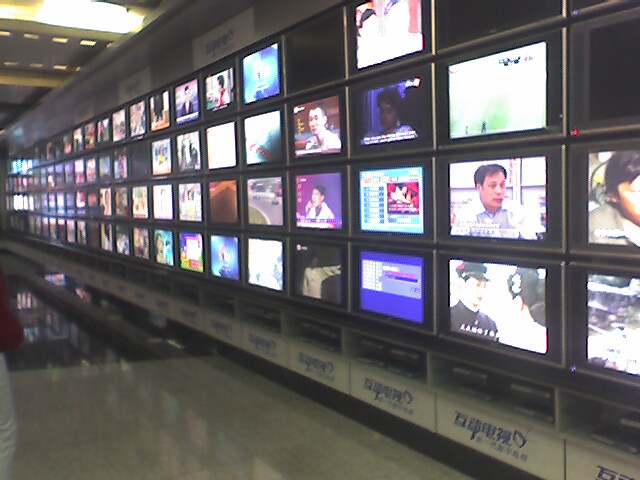The image depicts a section of a Chinese shopping mall with a tiled walking lane. Along one wall, there are four rows of old CRT (cathode ray tube) televisions, some of which are turned off or appear to have overheated or been damaged. The TVs are all the same size and display a variety of programs, including typical dramas, a steak show, Super Sentai or Power Rangers, racing, singing competitions, news reports, weather forecasts, and even some black-and-white shows. The scene is dimly lit, with the primary illumination coming from a single struggling fluorescent bulb in the upper left-hand corner. The lower section of the wall features white Chinese writing and some sort of cabinet beneath the TVs. The floor is composed of black and white tiles, creating a checkerboard pattern down the hallway.